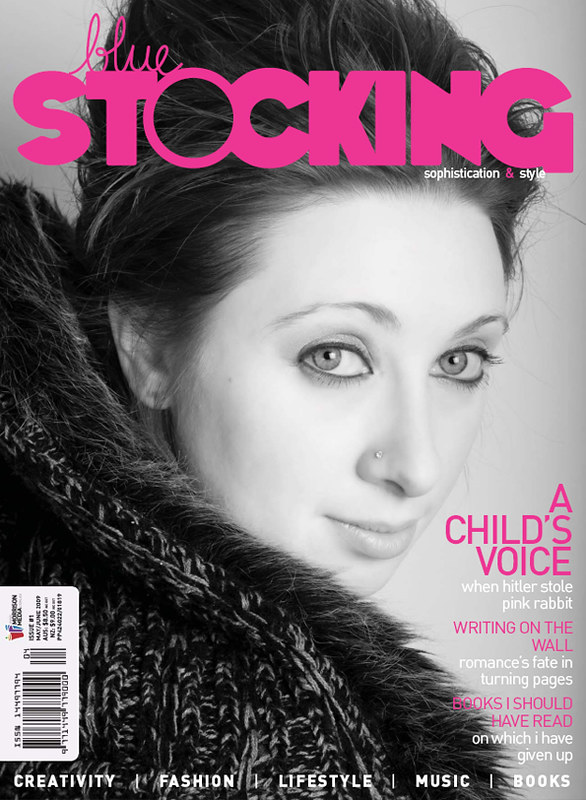The cover of the magazine "Blue Stocking" exudes sophistication and style. Featuring a striking black and white photograph, it showcases an attractive woman with brown hair styled in an updo, leaving the sides bare. Her grayish eyes and long, well-defined nose are accentuated by a diamond stud in one nostril. She is posing confidently in a thick fur coat. The cover highlights a mix of articles, with titles in both pink and white text. Featured articles include "A Child's Voice," "Books I Should Have Read," "Writing on the Wall," "When Hitler Stole Pink Rabbit," and "Romances Fade in Turning Pages." At the bottom, the categories of creativity, fashion, lifestyle, music, and books are listed in white text. A barcode on the left-hand side completes the cover layout. The overall composition emphasizes a blend of elegance and intellectual depth.